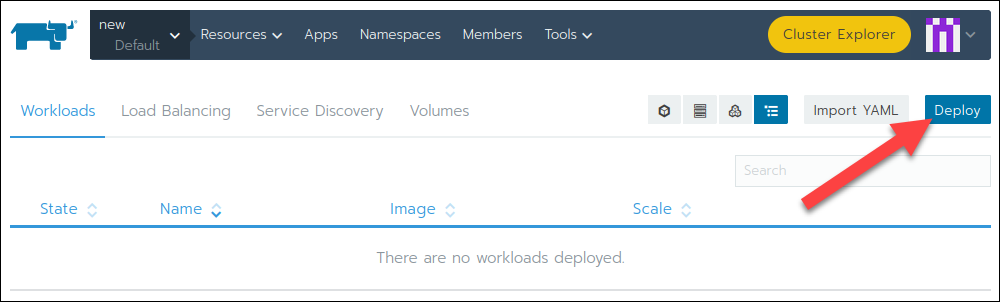This is a website with a white and blue color scheme. In the upper left-hand corner, there is a blue logo, resembling a bull, composed of square and rectangular shapes. To the right of the logo, "New" is displayed, followed by a dropdown labeled "Default." Next, there are several menu items: "Resources" with a dropdown arrow, "Apps," "Namespaces," "Members," and "Tools," which also has a dropdown arrow.

To the far right, highlighted in yellow, is "Cluster Explorer," and next to it, there's a white and purple logo that looks like a present box or a building, also with a dropdown arrow. Below this menu bar, a section is hyperlinked and highlighted in blue, labeled "Workloads." In gray, there are additional menu items: "Load Balancing," "Service Directory," and "Volumes."

To the right of these items, there are three gray symbols and one blue symbol, next to which the text "Import YAML" is displayed, followed by a blue button labeled "Deploy." Below this section, column headers include "State," "Name," "Image," and "Scale," each with up and down arrows for sorting. Currently, no workloads are deployed.